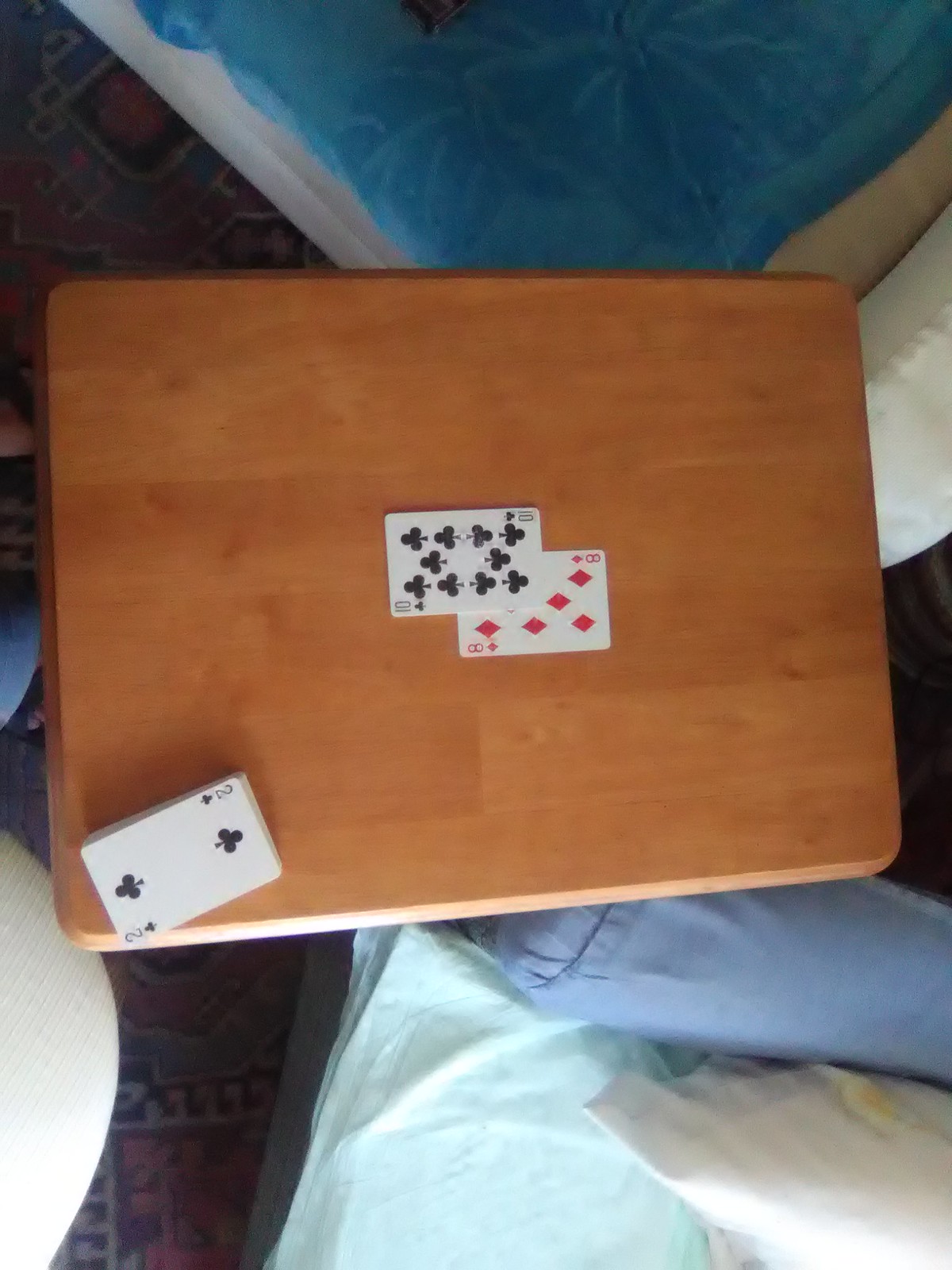In this slightly vertical photograph, a light brown table is positioned horizontally across the center, creating a cozy scene suggestive of a residence or camper interior. The tabletop hosts a deck of cards, with two cards—the eight of diamonds and the ten of clubs—prominently displayed in the center. The ten of clubs slightly overlaps the upper left quadrant of the eight of diamonds, both oriented horizontally. The remaining deck, with the two of clubs visible on top, sits slightly turned in the lower left corner of the table.

Surrounding the table are two sofas adding to the inviting atmosphere. At the top of the image, a white sofa features a blue towel draped over one of its cushions. Below the table, another sofa in a lighter denim blue hue is adorned with a white pillow and a green towel, further enhancing the cozy, lived-in feel of the space. The overall composition of the scene evokes a sense of relaxation and casual leisure.